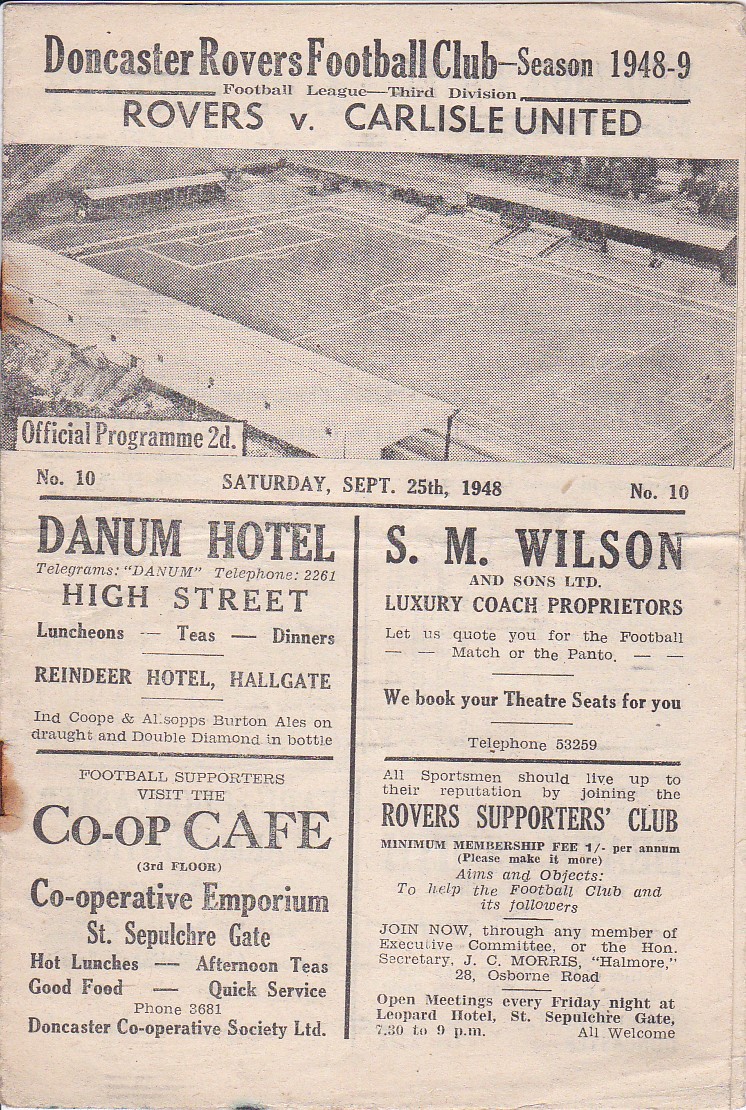The image depicts a retro-style advertisement or program from the Doncaster Rovers Football Club's 1948-49 season. The yellowed paper features a prominent title at the top, “Doncaster Rovers Football Club Season 1948-49,” followed by "Rovers vs. Carlisle United." A large black-and-white photograph of a football field spans the paper’s width beneath the title. The text “Official Program 2D” is located in the bottom right corner of the image. Centered beneath the photo are the words “Saturday, September 25th, 1948,” with a black horizontal line running underneath. The bottom section of the image is populated with various advertisements. On the right, there is an ad for “S.M. Wilson and Sons Limited, Luxury Coach Proprietors,” and the Rovers Supporters Club information follows below. On the left, under the date, an ad for “Danum Hotel, High Street” is presented, with mentions of “Luncheons, Teas, Dinners,” and the “Reindeer Hotel, Hallgate.” The bottom left features the “Co-op Café,” located on the third floor of the Cooperative Emporium at St. Sepulchre’s Gate. The program’s colors include shades of tan, white, black, and gray, emphasizing its vintage feel.